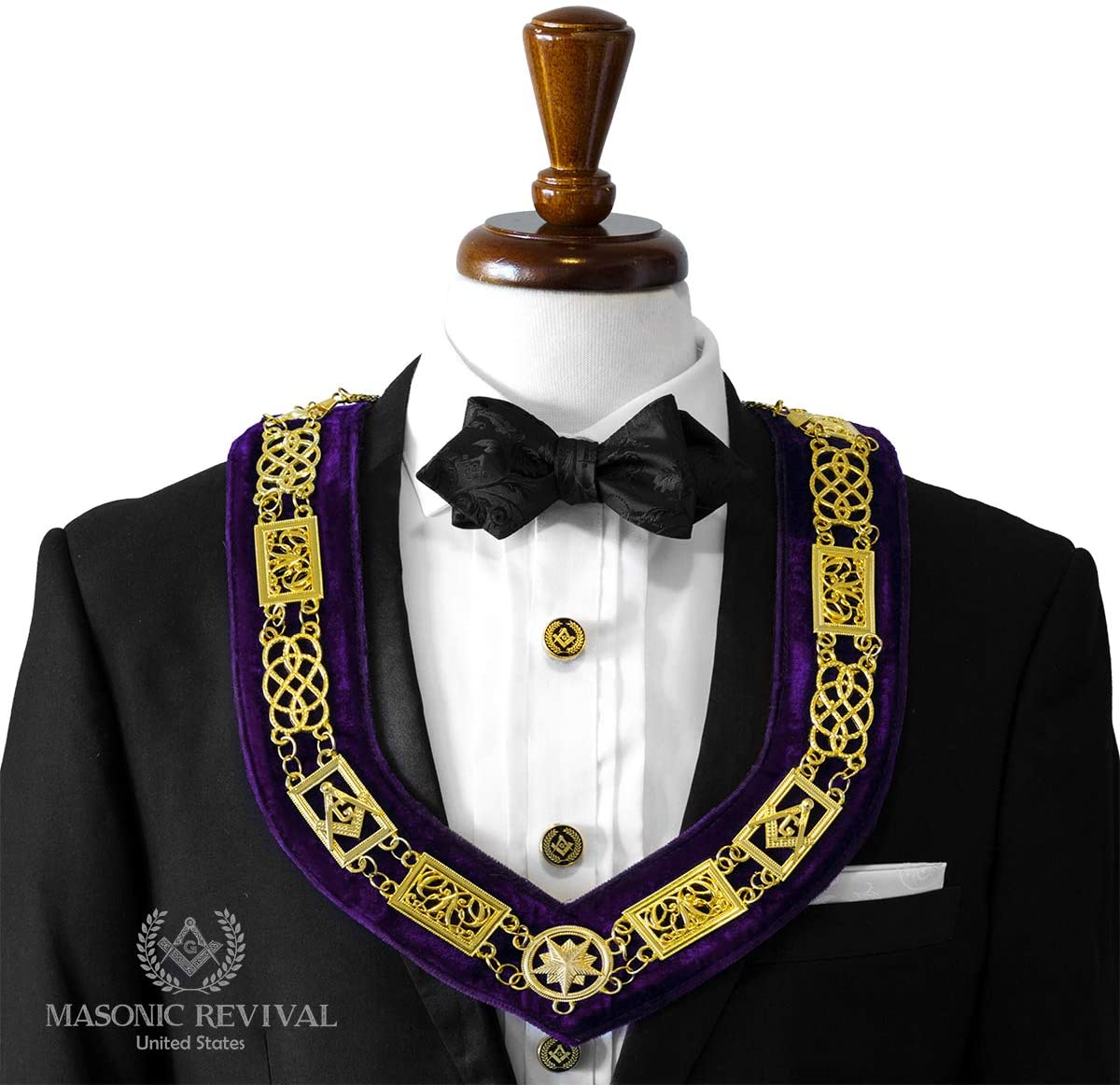This photograph features a headless mannequin dressed in an ornate Masonic outfit. The ensemble includes a black tuxedo jacket, a crisp white dress shirt adorned with three distinctive Masonic buttons, and a black bow tie. Draped over the mannequin's shoulders and cascading down to the lower chest area is a luxurious purple velvet sash trimmed in gold, decorated with a series of rectangular emblems and chain-link designs, culminating in a Masonic emblem at the tip. A white handkerchief neatly peeks out from the jacket's pocket. The image bears the inscription "Masonic Revival United States" in the bottom left corner, reinforcing the ceremonial and historical significance of the attire. The mannequin's neck area features a wooden dowel, indicating it is deliberately headless for display purposes.